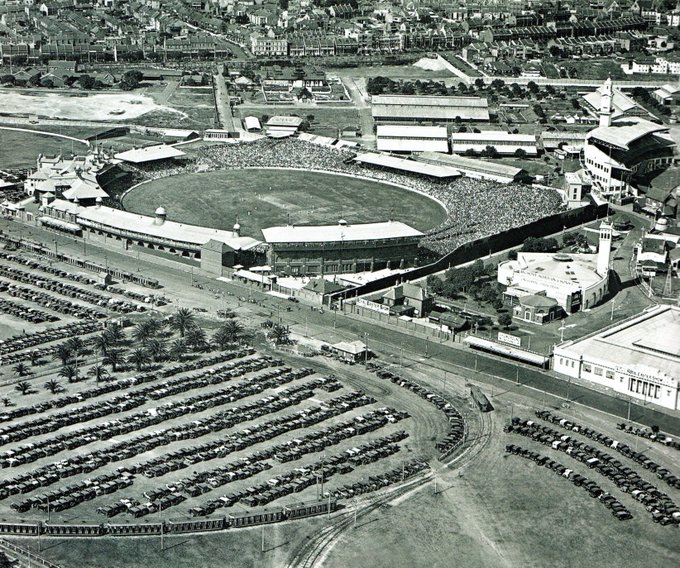This vintage black-and-white photograph showcases a bustling scene of a large town or city during the early 20th century. The focal point of the image is a grand, circular sports field, likely a cricket or rugby stadium, situated in the upper half of the square photo. The stadium is filled with countless spectators, indicating an ongoing sports event. Surrounding the stadium are various buildings, including warehouses and residential row houses.

Running diagonally from the middle left to the lower right of the image, a prominent road separates the stadium area from a vast parking lot, which is also circular in shape and packed with numerous, distinctively old cars, resembling Model Ts. This detailed aerial view, possibly captured from a drone or aircraft, provides a comprehensive glimpse into a bygone era, showcasing the architecture, infrastructure, and lively atmosphere of the time.